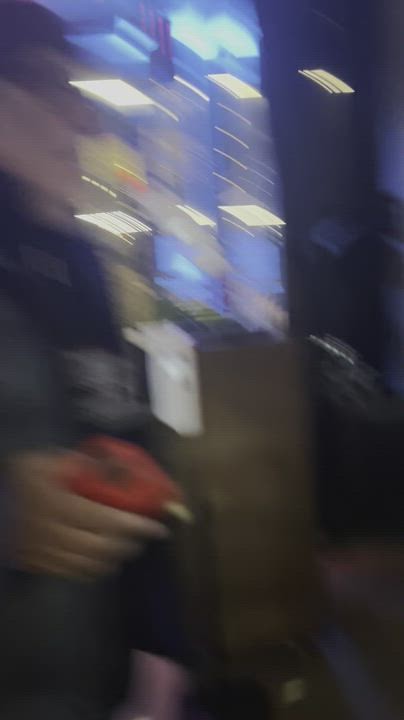In this incredibly blurry vertical iPhone shot, a person with a long sleeve shirt, possibly wearing a cap or hat, stands on the left side of the image. The person, who might be a woman with glasses, holds something red in their right hand, potentially a tomato or a pepper. They are wearing a black uniform with an unreadable text on it and have a ring, possibly a wedding band, on one finger. The background features darkened surroundings with illuminated glass windows and office lights creating reflections, suggesting an indoor setting. Objects such as boxes can be faintly seen at the bottom, adding a textured element to the otherwise fuzzy and out-of-focus scene.